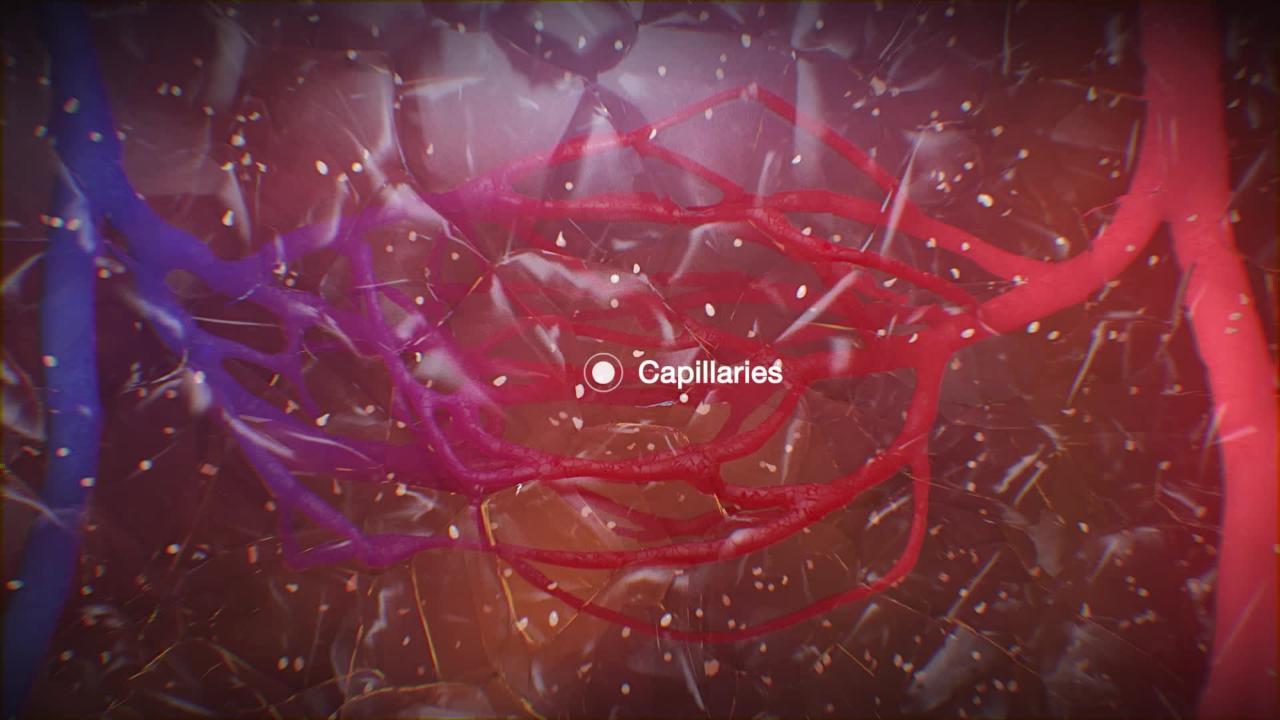This image is a computer-generated graphic depicting capillaries within the human body. The background predominantly features shades of red, blue, and purple, suggesting the various states of blood oxygenation—red for oxygen-rich blood from the heart and blue for oxygen-depleted blood returning to the heart. The whole image is structured as a horizontal rectangle, approximately twice as wide as it is tall, with the label "capillaries" in white text centrally positioned. Immediately to the right of this word is a solid white dot encircled by a white ring.

The visual showcases a complex network of capillaries branching out horizontally from larger vertical veins located on the left and right edges of the image, converging towards the center. Adding to the detail are numerous white flecks scattered across the graphic, possibly indicating specific highlighting points or artistic embellishments. The background itself has a maroon or reddish-brown hue, implying an underlying muscle or tissue context, further enriched by shadowing effects that give a sense of depth and texture. Overall, this composite serves as a detailed illustration of the capillary system, enhanced by artistic elements to portray its intricate nature.